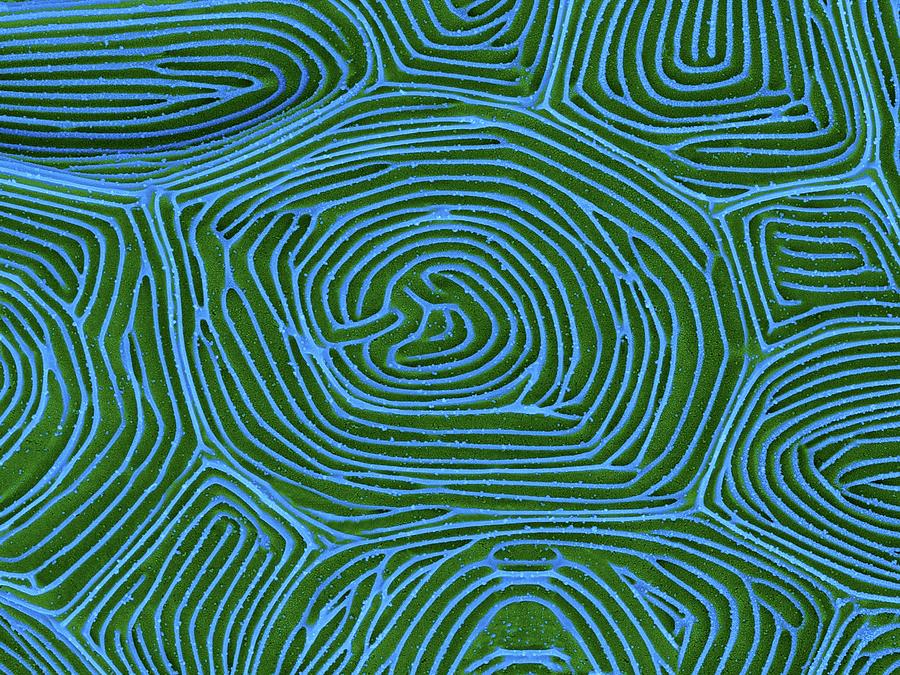The image is a mesmerizing abstract design, possibly a painting or drawing, featuring a central shape with an intricate pattern. The pattern consists of concentric, maze-like blue lines interspersed with green, forming a visual effect reminiscent of a sliced clove of garlic dyed in vibrant colors. This central motif, marked by its light blue and green lines, is surrounded by nine similarly designed shapes of varying sizes, creating a harmonious and symmetrical layout. The overall impression is one of a beautiful, yet ambiguous abstraction that could be interpreted as an aerial view of a green landscape with sparkling, blue swirls, highlighting the delicate interplay between order and variation.